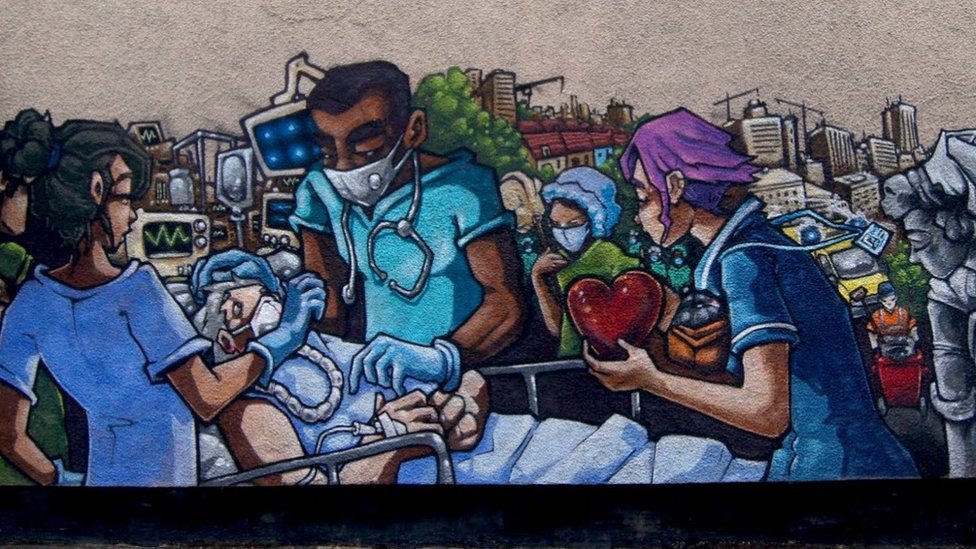The image depicts an intricate and poignant painted scene of an emergency medical situation, rendering a blend of indoor and outdoor settings. Central to the composition is a person lying in a gurney, equipped with a white oxygen mask. Surrounding the patient are three medical professionals: a doctor, distinguishable by a stethoscope and mask, and two nurses, one of whom holds a red heart in her hand. This evocative detail hints at the urgency of a possible heart transplant scenario. The attire of the figures ranges from blue to purple, adding a somber yet vibrant contrast to the scene.

In the background, there is an intriguing dichotomy—the left side and top are enclosed by a beige wall adorned with various medical equipment and computers, indicative of a hospital environment, whereas the right side expands into the bustling urban landscape of downtown Atlanta, complete with city buildings, green trees, and a gray sky. The onlookers in the background, all wearing masks, add to the sense of a critical and communal moment.

The visual composition elegantly blends the sterile hospital ambiance with the dynamic cityscape, symbolically representing the 'heart of the city' and highlighting the collective concern for the patient's wellbeing.